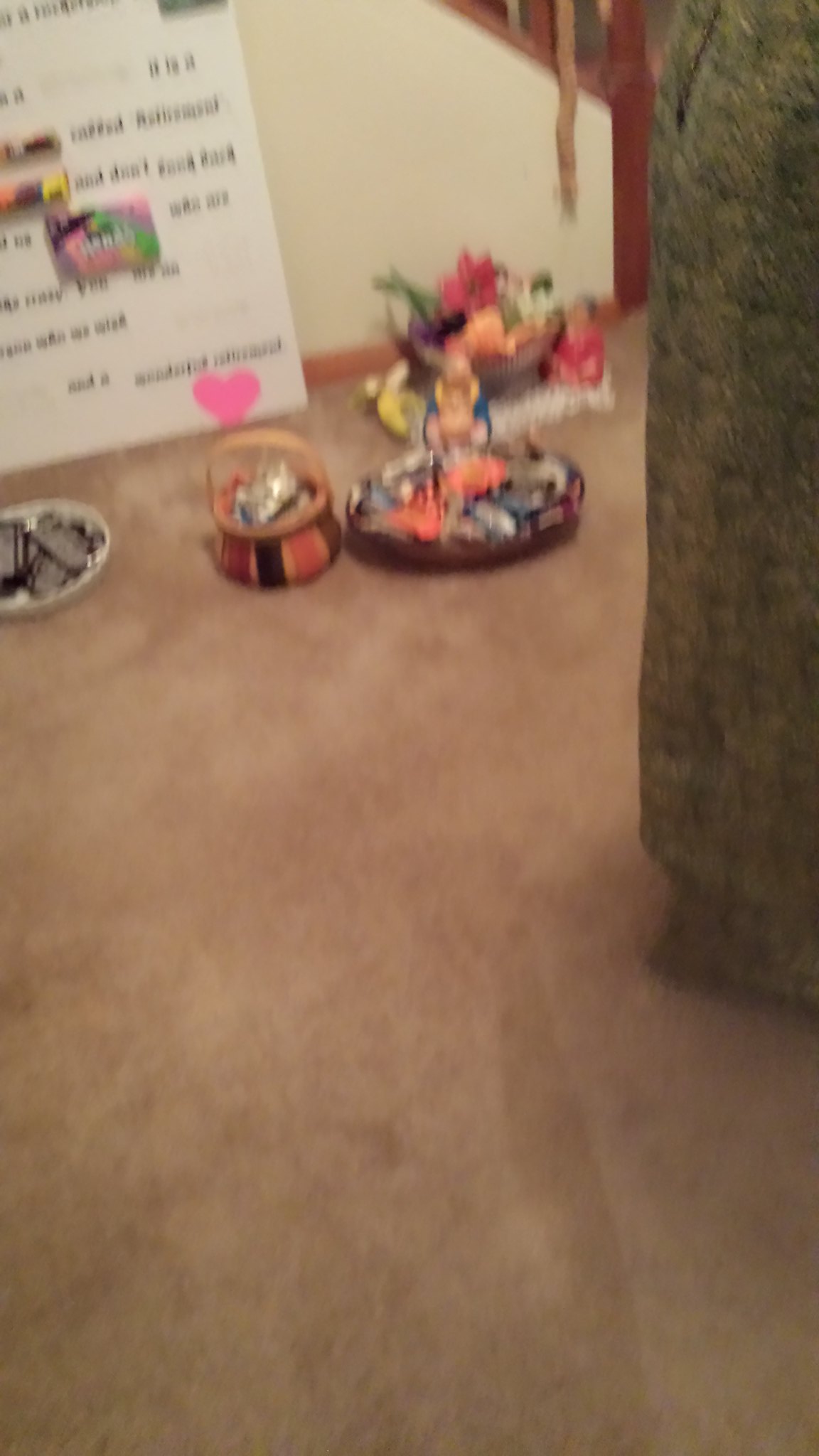The image depicts a scene with multiple baskets and plates arranged on a light brown carpeted floor. The scene includes a variety of colorful objects, likely candies or confectioneries, and possibly flowers. There is a prominent white sign in the background adorned with black lettering and multicolored decorations, including candies taped on to form words or enhance the message. A distinct pink heart can be seen on the lower right-hand corner of the sign. Towards the right side of the image stands a tall, tube-like, grayish-green structure, possibly made of cloth. The floor arrangement includes a white plate with chocolates, a beige and pink basket with wrapped sweets, and a large open basket with a handle, containing red and brown items. Another basket features pink and white flowers. The setting includes a staircase in the background, adding depth to the scene. The overall collection appears to be meticulously arranged, potentially as a gift display.